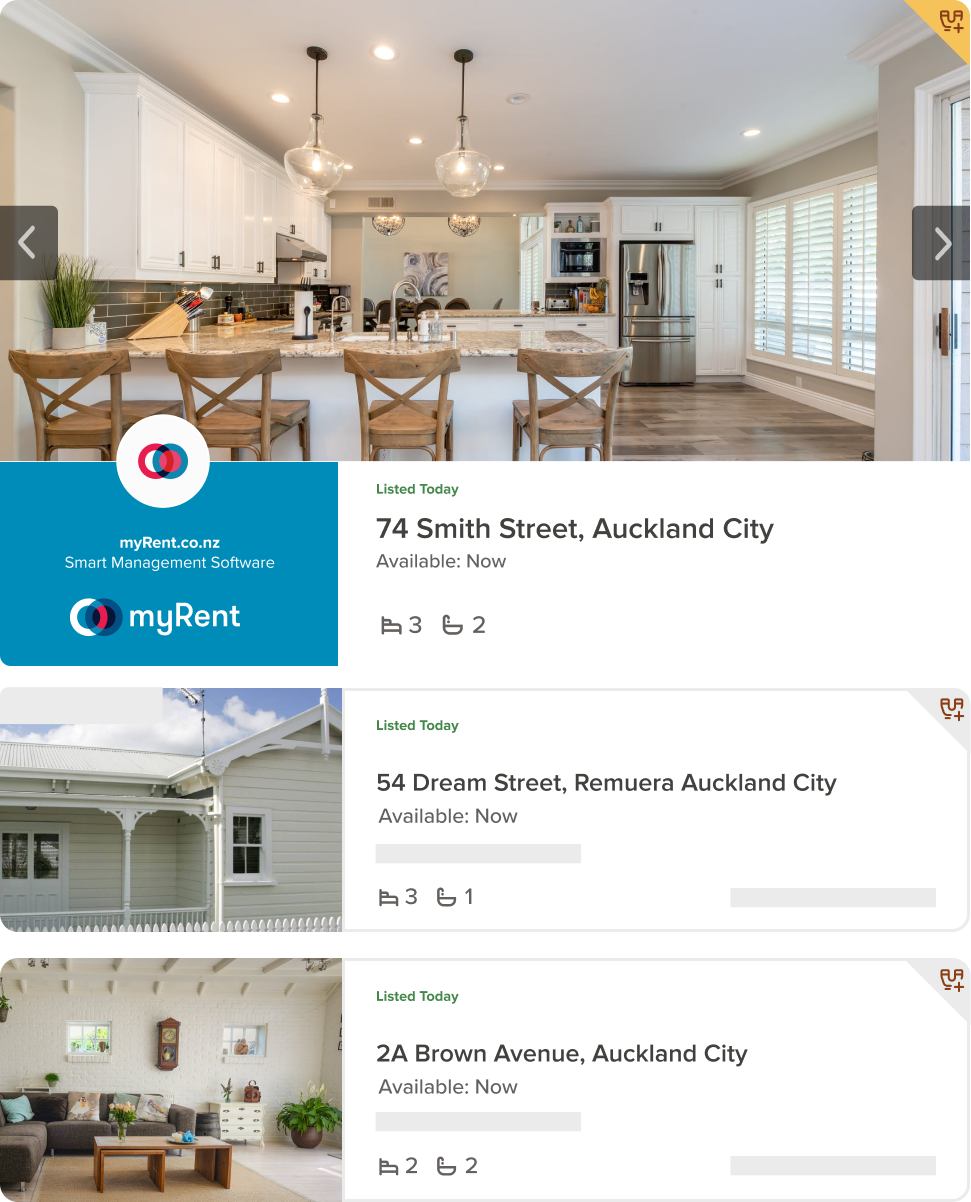A screenshot from a rental company's website showcases a search result displaying available properties in Auckland City. The top section features a large image of a modern kitchen with an open layout. The kitchen includes a stainless steel fridge, a marble or granite countertop that serves as an island with four chairs, and a sidebar where meals can be enjoyed while looking into the kitchen space. The featured property is listed as "74 Smith Suite," and is currently available for rent. It offers three bedrooms and two bathrooms, as indicated by respective icons. The property's details are followed by a blue box displaying the website myrent.co.nz, which promotes its smart management software with a logo featuring red, white, and gray colors.

Below the primary listing, two additional properties are shown: one located at "54 Dream Street" and another at "2A Brown Avenue," both also situated in Auckland City. Each listing includes a small corresponding image, providing potential renters with a quick visual reference of the properties.